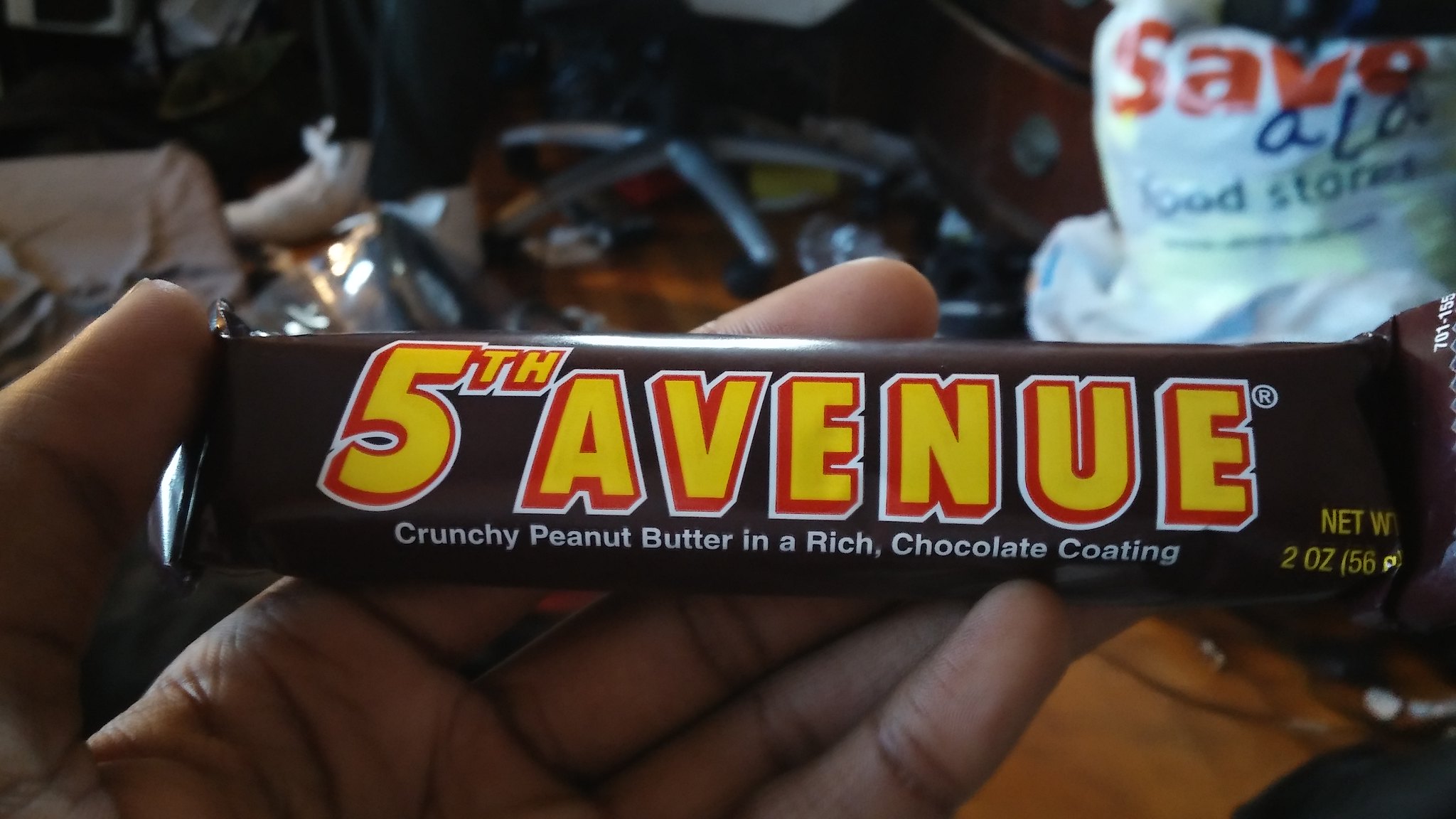This is a close-up photo capturing a man's hand holding a brand-new 5th Avenue candy bar. The candy bar wrapper is dark brown with bold yellow letters outlined in red that read "5th Avenue." Below this, white text states, "crunchy peanut butter in a rich chocolate coating." Also visible on the wrapper, in smaller yellow font, is "net weight 2 ounces (56g)." The candy bar rests on the man's thumb and fingers, prominently positioned across the palm of his hand.

In the background, which is out of focus, there appears to be a cluttered room. Key identifiable items include a crumpled white plastic bag with the "Save-A-Lot Food Stores" logo displayed in red, blue, and green text, as well as the bottom of a silver rolling chair. Additionally, there are various indistinct objects and colors, including a notable white and orangey hue, contributing to the overall disarray.